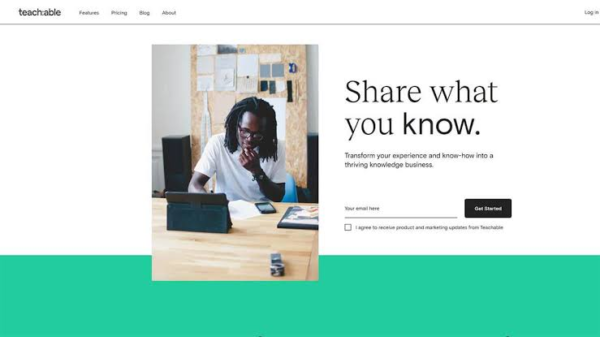The image appears to be a screenshot from a computer, formatted in a horizontal rectangular shape with a predominantly white background and black text. In the top left corner, the bold text reads "Teachable." Adjacent to this are clickable menu options: Features, Pricing, Blog, About, and on the far right, a Login button. Below this header is a thin black line, under which sits a centrally-left positioned photograph.

The photograph features a black man with long braided hair and glasses, seated at a desk and facing the camera. He is dressed in a white t-shirt with his left elbow resting on the desk, hands thoughtfully touching his chin. In front of him on the desk are several items: a piece of paper he appears to be writing on, a cell phone, and a tablet positioned upright, which he is looking at intently.

To the right of the photograph is a motivational prompt: "Share what you know. Transform your experience and know-how into a thriving knowledge business." Below this prompt is a field labeled "Your email here" and a button that says "Get started." The bottom portion of the image features a prominent green rectangular line.